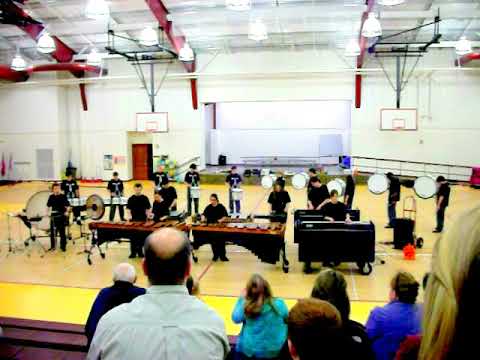In the photograph, we see a school gymnasium with a polished wooden floor and basketball hoops folded up against the back wall. Overhead, large gymnasium-style lights hang from the ceiling, illuminating the scene. To the left of the wall in the background, there's a small red door and possibly a stage area. 

Centered in the gymnasium is a marching band ensemble. The group includes various percussion instruments: a large xylophone table played by two or three people in front, numerous drums of different sizes handled by about eight individuals in the back, a person with a pair of cymbals, and a keyboard player positioned to the right. All band members are wearing black shirts.

The image is taken from the bleachers, capturing the backs of a few spectators who are watching the band's performance. The bleachers run along the left side of the image, providing a vantage point that highlights the school's gym setting. The color palette of the photograph includes purples, yellows, light blue, black, tan, dark blue, white, and gray, adding vibrancy to the detailed indoor scene.